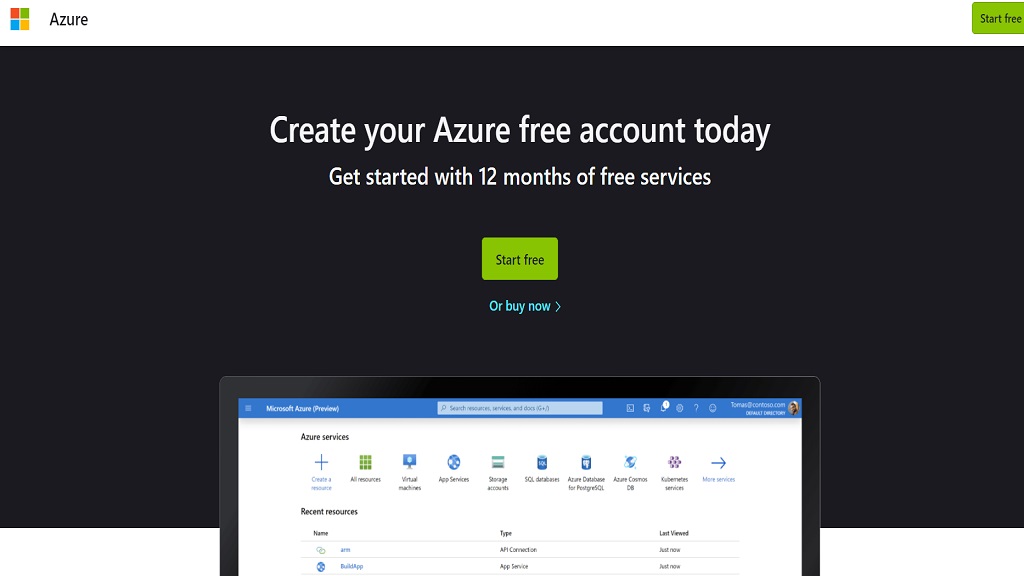In this image, the primary focus is a Microsoft Azure webpage encouraging users to create a free account. Prominently displayed at the top is a bold headline: "Create Your Azure Free Account Today." The offer includes 12 months of free services, which is emphasized further by two call-to-action buttons: "Start Free" and "Buy Now." The "Start Free" button is notably positioned in the top right corner of the page for easy access.

Beneath the headline, the page features an embedded image of a tablet screen showcasing various Azure services. The screen displays text labels such as "Azure Services," and "Microsoft Azure Preview." A search bar is visible for quick navigation, along with user account information located at the top right of the tablet interface. 

Additionally, various service categories are listed, including "Create a Resource," "Virtual Machines," "App Services," "Storage Accounts," "SQL Databases," and "Azure Database for PostgreSQL." These elements highlight the extensive and versatile functionalities available through Microsoft's Azure platform.